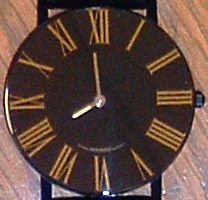The image depicts a watch with a chocolate brown face, adorned with Roman numerals painted in a tan or yellow hue. The face of the watch is circular, contained within a metallic frame, and appears to be sitting on a wooden countertop that matches the brown tones of the watch face. The Roman numerals are evenly spaced around the dial, starting with 'XII' at the top and progressing clockwise until 'VI' at the bottom. The time displayed is approximately 7:58, with the minute hand almost at 'XII' and the hour hand near 'VIII'. The watch features a reflective, possibly illuminated hour hand, contrasting with the non-illuminated minute hand, both seemingly made of a golden metallic material. Additionally, on the right side of the watch, there is a small winding dial used to adjust the time. The overall image is described as a tiny square, capturing the detailed and elegant design of the watch against a wooden backdrop.